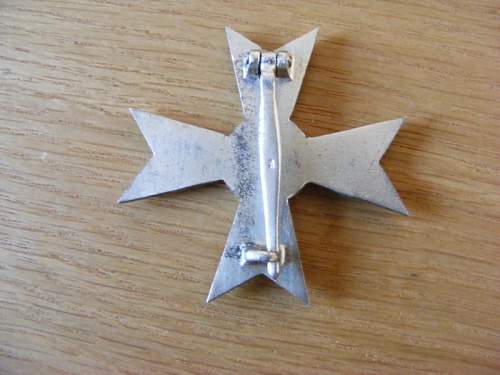The image features a single metal object, likely a piece of jewelry such as a brooch or pin, positioned slightly off-center on a wooden surface, which might be a desk or a table. The wood grain of the background angles downward to the right at about 20 degrees, providing a natural, rustic setting in contrast to the sleekness of the metal piece. This metal object, possibly made of silver or pewter, is displayed upside down, showcasing the backside which includes the clasp mechanism. The object consists of a circular center with four notched arms extending towards the north, south, east, and west, each forming a wide V shape at the ends. The clasp runs along the north and south arms, while the east and west arms remain unclasped. The metal appears somewhat burnished, indicating it may have been hammered out during its creation. The arrangement draws the viewer’s eye towards the metallic luster and intricate design of the piece against the contrasting wooden backdrop.